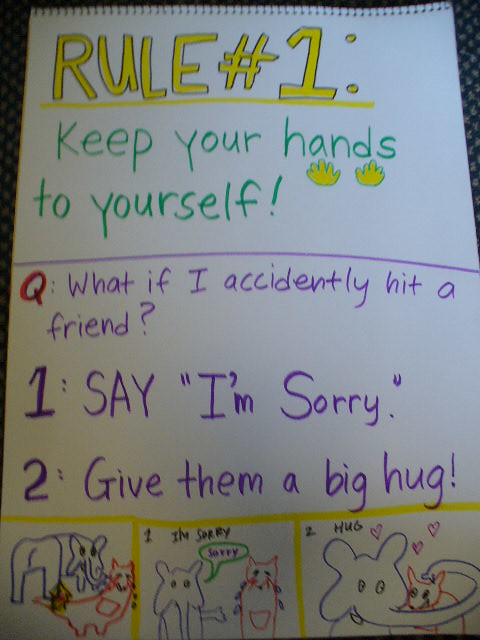This image showcases a large, white, hand-drawn poster that illustrates a set of rules for handling accidental conflicts among friends. At the very top, in yellow writing outlined by black, it boldly states "Rule Number One: Keep your hands to yourself," accompanied by a child-like drawing of two hands. Below this, written in purple marker, is the question, "What if I accidentally hit a friend?" followed by two steps: "1. Say I'm sorry," and "2. Give them a big hug." These steps are visually depicted in a three-part cartoon storyboard beneath the text. In the first panel, an elephant is shown accidentally hitting a smaller animal, potentially a cat or a fox. The second panel illustrates the elephant saying "I'm sorry" in a speech bubble, while the final panel depicts the elephant using its trunk to give the smaller animal a hug, symbolizing reconciliation and renewed friendship.